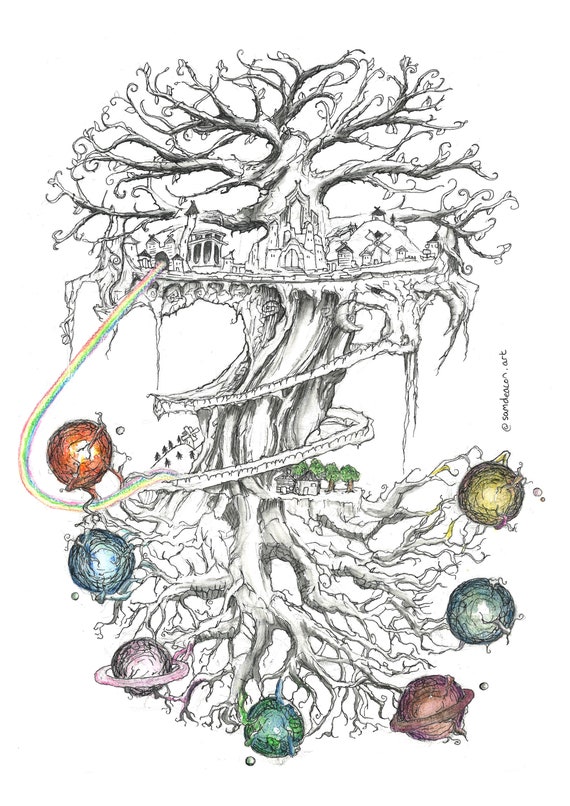The image is a detailed fantasy illustration presented in a vertical-rectangular format with no discernible border. Dominating the scene is an enormous, surreal tree, entirely devoid of leaves. The tree stretches upwards to reveal bare branches at the top and extends downwards into a subterranean view of its roots. The illustration appears to be a cross-section, enabling a clear view of both the surface and underground levels.

Perched among the lower branches of the tree is a treehouse complex, encompassing multiple structures and giving off an air of otherworldly architecture, possibly resembling a palace. A ramp spirals elegantly from the base of the tree up to this treehouse, accompanied by what appears to be an exit chute descending from the treehouse down to the roots.

The base of the tree reveals a fascinating underground network where several colored spheres, reminiscent of planets or satellites, are intertwined with the roots. The seven spheres vary in vibrant hues, including red, blue, purple, dark blue, dark purple, light green, and yellow. Additionally, a rainbow arcs from the treehouse downwards, intersecting with a sandy area below, which is dotted with green trees. Contrasting these vibrant elements, the rest of the tree and the background are rendered in striking black and white, enhancing the fantasy aspect of the illustration.